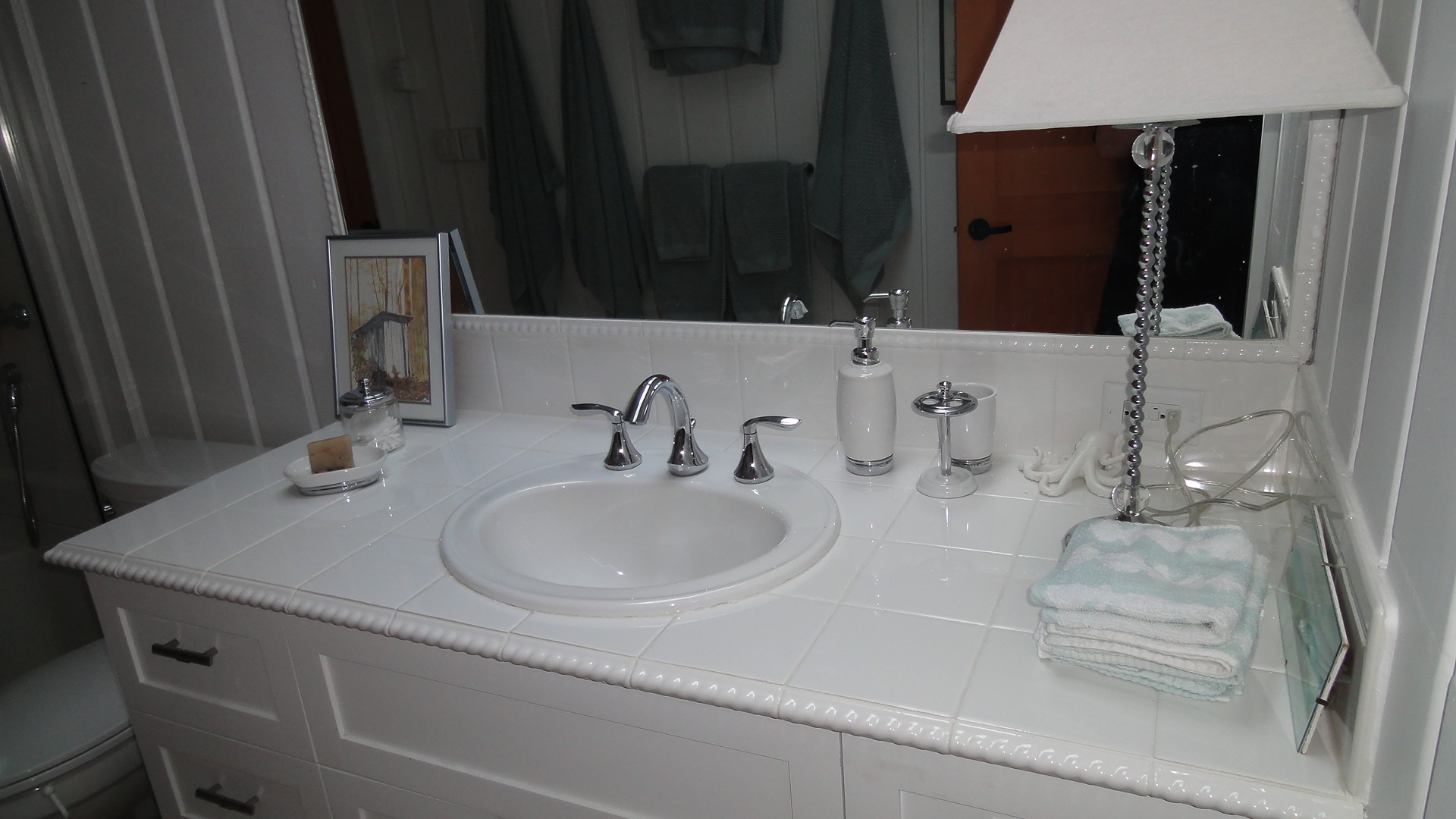In the image of the bathroom, the scene is centered around a pristine white countertop. Prominently featured on the countertop is a sleek, white basin, accompanied by a silver metal faucet with dual handles. Positioned just behind the basin, there is a white soap dispenser topped with a metal tube. To the immediate right of the dispenser stands a small, white cup, and adjacent to it sits a quirky white octopus-shaped object. Nearby, an electrical cable is plugged into an outlet on the wall.

Further to the right, the bottom portion of a lamp is visible, with the lampshade atop it. In front of the lamp lies a neatly stacked pile of face towels accompanied by a small, unidentifiable picture or object. The white wall to the right contrasts with these items.

On the left side of the basin, a picture frame displaying an image of trees rests on the countertop. Next to the frame, there is a small jar and a tray holding a brown bar of soap. Beneath the sink, white drawers can be seen. The wall to the left houses a toilet, and reflected in the mirror are blue towels hanging on the wall and a brown door in the background.